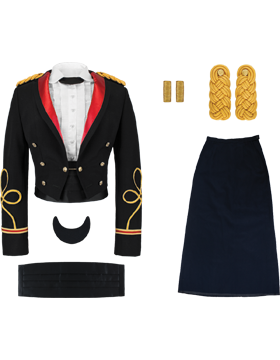The image displays a woman's formal uniform meticulously laid out in its individual components against a stark white background. The primary piece is a dark jacket, which is intricately designed with gold embroidery, gold buttons, and elaborate embellishments. The sleeves of the jacket are adorned with a red and gold trim, featuring ornate gold embroidery that resembles bows or flowers. The lapels are lined with luxurious red satin or silk, adding a touch of elegance.

Prominently displayed on the shoulders of the jacket are gold epaulets or amulets, indicative of a rank, though the specific type of uniform—whether military or ceremonial dress attire—remains unclear. Complementing the jacket is a long, dark skirt, either black or navy blue, which suggests the uniform might be intended for formal occasions. In addition, there is a black belt laid out beneath the jacket, and a pair of yellow, woven items with small holes at the top, possibly part of the decorations worn on the uniform's shoulders. Adjacent to these, there are two smaller yellow rectangular items, possibly additional embellishments or insignias. Overall, the ensemble appears to be a formal dress uniform for a woman, characterized by its detailed and elegant design.